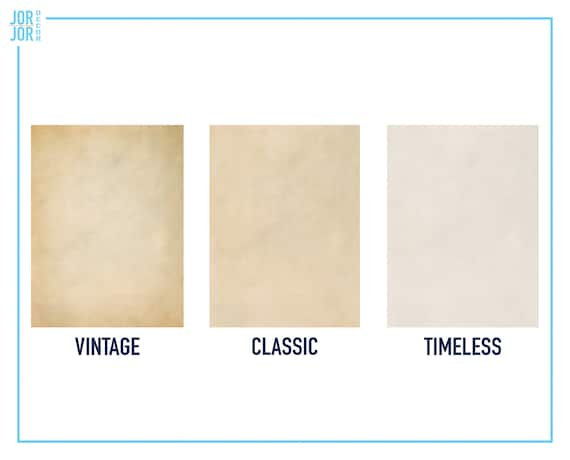The image displays a white background with a square-shaped, light blue border featuring the name "Jor Jor" in the top left corner. Inside the square are three distinct options for couch colors, each represented by squarish colored boxes with bold text beneath them. From left to right, the first box is a beige-pink hue labeled "Vintage," appearing as the darkest among the options. The middle box is a tan or pinkish-lavender color, described as "Classic," and represents a medium shade. The final box on the far right has a cream or mostly lavender color, labeled "Timeless," and is the lightest of the three. All the colors share a brownish, cream, or tan aesthetic, offering a cohesive, yet subtly varied palette for couch selection.